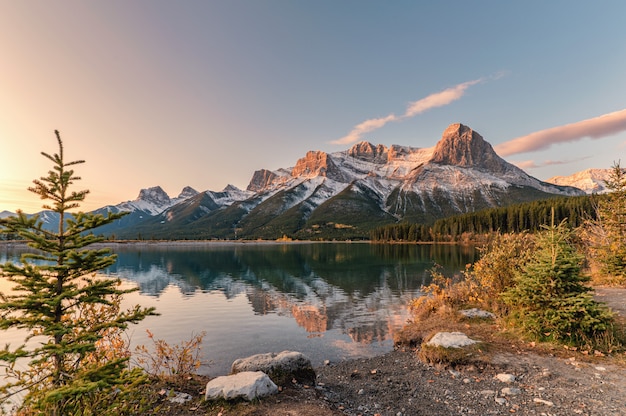The image captures a serene and picturesque outdoor scene during the daytime, likely taken near sunrise, suggested by the bright illumination on the left-hand side. Dominated by a clear blue sky with minimal clouds primarily on the right, the photograph showcases a tranquil mountain lake bordered by snow-capped peaks that stretch horizontally from right to left across the background. The lake's still, unpolluted green waters mirror the rugged, snow-touched mountains, enhancing the natural beauty of the landscape. In the foreground, a Christmas-like pine tree stands prominently on the left, while a patch of gravel and dirt occupies the space directly in front of the lake, possibly leading to a swimming area. The right side of the image is densely populated with trees, resembling a forest. There are no people or animals visible, which adds to the undisturbed and pristine quality of the scene. The overall composition, likely intended for a photography portfolio, is both detailed and artful, capturing the essence of an untouched natural environment in what appears to be late spring, around April or May.